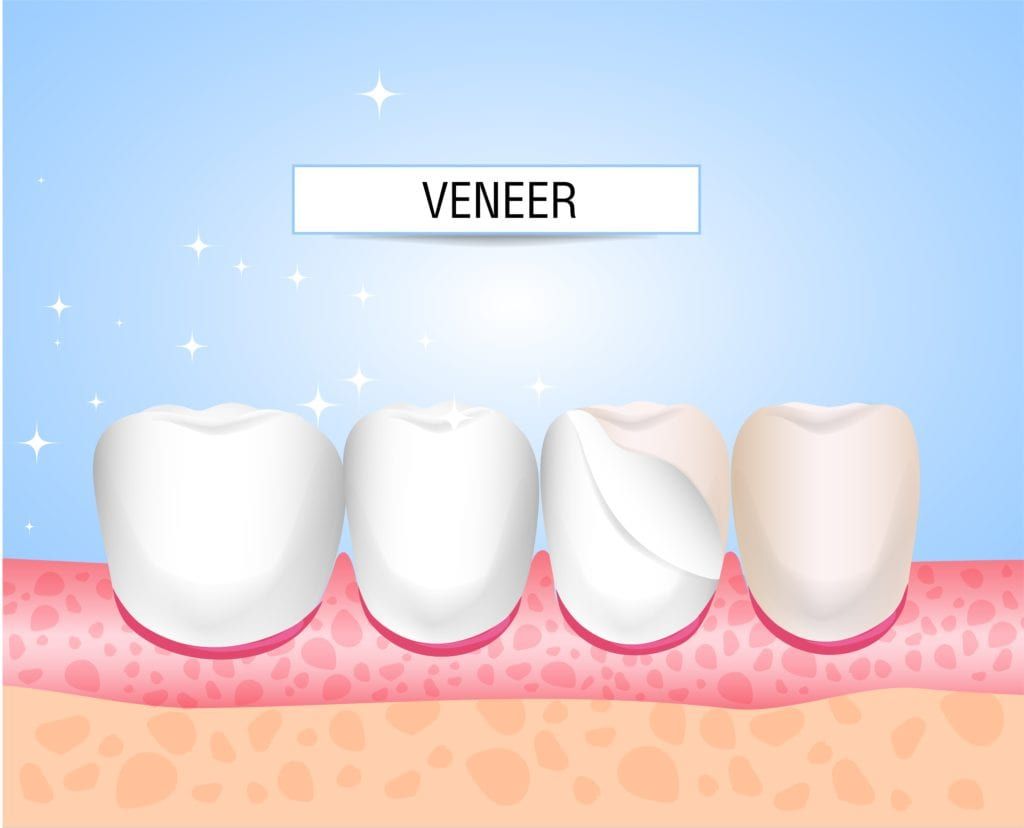The image is a computer-generated graphic with a light sky blue background scattered with white stars. At the top center, a thin rectangular white banner with a blue border displays the word "VENEER" in all capital black letters. Below the banner, the main focus is on a depiction of four teeth set into pink gums. The teeth, stylized as ovals with slightly inward-curving tops, are positioned above a light orangish-pink wavy stripe with darker circles, representing a simplified layer of skin beneath the gums. The first two teeth on the left are covered by white veneers, which sparkle to emphasize their brightness, while the third tooth shows the veneer partially peeled back to reveal the yellowed tooth underneath. This visual contrast highlights the transformative effect of veneers.